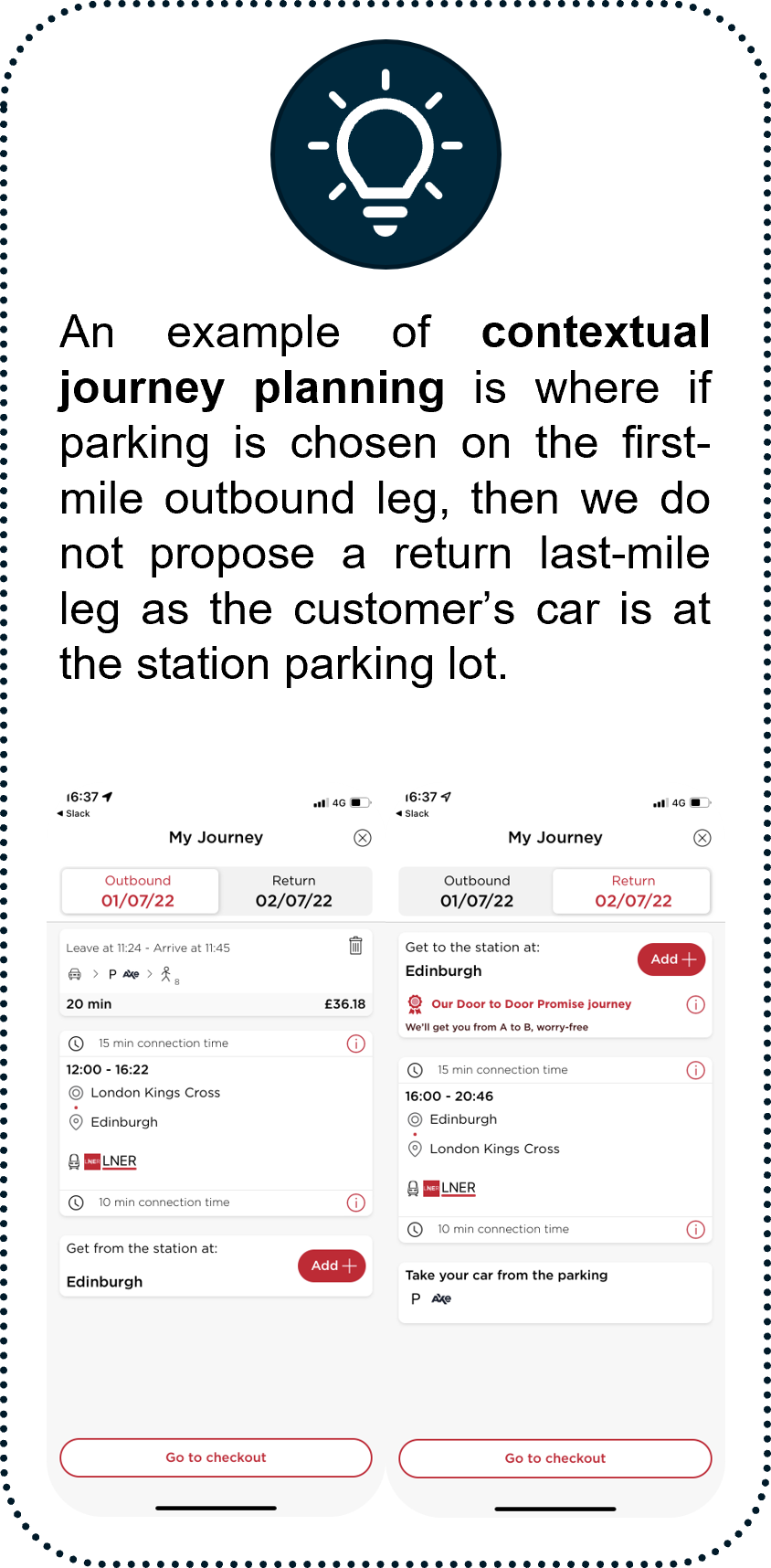A prime example of contextual journey planning is demonstrated in this image, where selecting parking for the initial outbound leg negates the need to propose a return last-mile leg, as the customer's car remains at the station's parking lot. The journey begins with an outbound leg from 107.22 to 207.22, lasting 20 minutes from 6:18 to 6:22, departing from London Kings Cross and arriving at Edinburgh on the LNER service. There's a 10-minute connection time requirement at Edinburgh Station. The return journey starts from 107.22 and ends at 207.22, ensuring a worry-free door-to-door travel experience, facilitated by our promise of seamless transitions. The return trip also includes a 15-minute connection from 16:00 to 20:46, traveling from Edinburgh back to London Kings Cross on the LNER service, again featuring a 10-minute connection time. Upon arrival, customers can retrieve their cars from the parking lot, indicated by the "P" sign, and proceed to checkout. The image itself is bordered by a dotted line and features a light bulb at the top, symbolizing innovative and illuminated travel solutions.